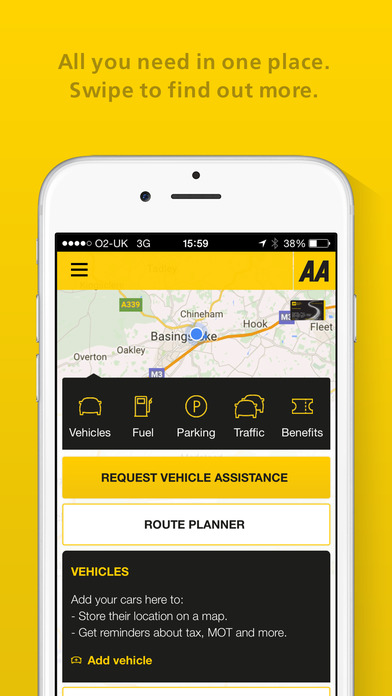This is a screenshot of an advertisement with a vibrant yellow background. At the top of the image, there is grayed-out text stating, "All you need in one place." The focal point at the bottom is a white smartphone displaying a detailed screen. The screen indicates the time as 15:59 and the battery percentage at 38%. In the top left corner, the text "O2 UK" suggests the phone is connected to the O2 network in the United Kingdom. The smartphone screen shows a map highlighting a location in Basingstoke, UK.

Below the map, several options are listed: "Vehicles," "Fuel," "Parking," "Traffic," and "Benefits." A prominent yellow button with black text offers the option to "Request Vehicle Assistance," while a white button below it is labeled "Route Planner." Further down, a section titled "Vehicles" invites users to "Add your cars here to store their location and get reminders about tax MOT and more." At the very bottom, there is a button to "Add Vehicle."